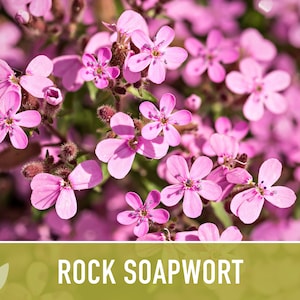The image captures a bush of Rock Soapwort flowers, displaying an array of pink to light purple blooms each with five oval petals arranged in a slightly star-like fashion. Among the blossoms, some flowers remain as unopened bulbs. The photograph possesses a low-quality, slightly blurry aesthetic, particularly noticeable in the green and pink background. The flowers feature distinct black dots at the tips of the petals and some have a mysterious growth in their centers. The text "ROCK SOAPWORT" is prominently overlaid at the bottom of the image on a semi-transparent green bar bordered in white, ensuring the flowers are still partially visible through the background.